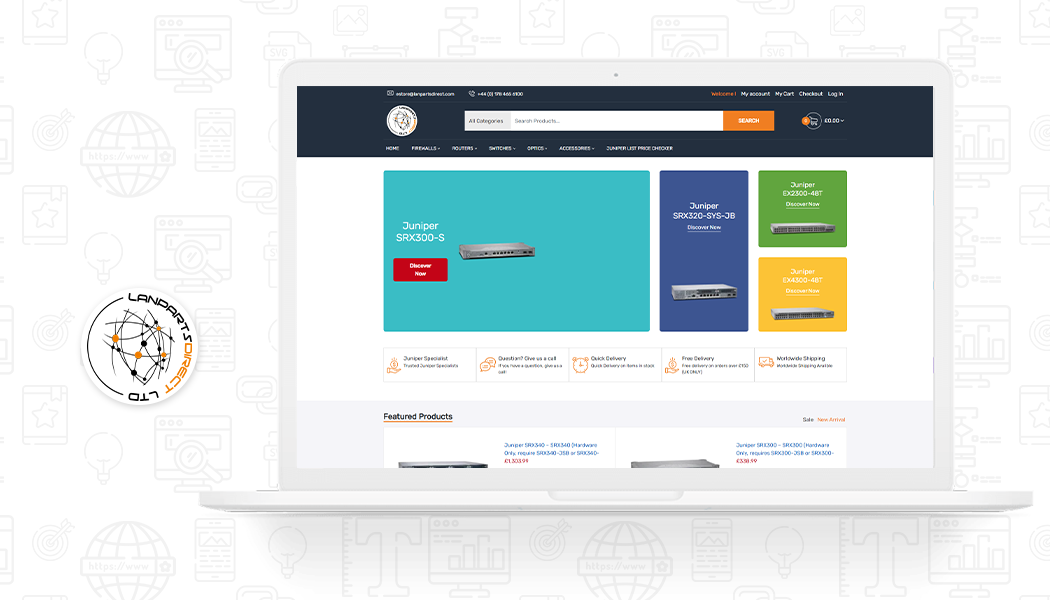The screenshot displays the homepage of Lands Parts Direct Limited, a website specializing in electronic equipment. The most prominent section features four distinct colored boxes highlighting various Juniper electronic products. The largest box, colored turquoise, showcases the Juniper SRX 300-S. To its right, the second largest box in blue promotes the Juniper SRX 320-SYS-JB. Adjacent to these, there are two smaller boxes; the green one features the Juniper EX-2300-48T, while the yellow box below displays the Juniper EX-4300-487. Each product box includes clear labeling, with some text being slightly harder to read due to smaller font size. The arrangement of boxes creates a visually structured layout, emphasizing the variety of Juniper electronics available for purchase.